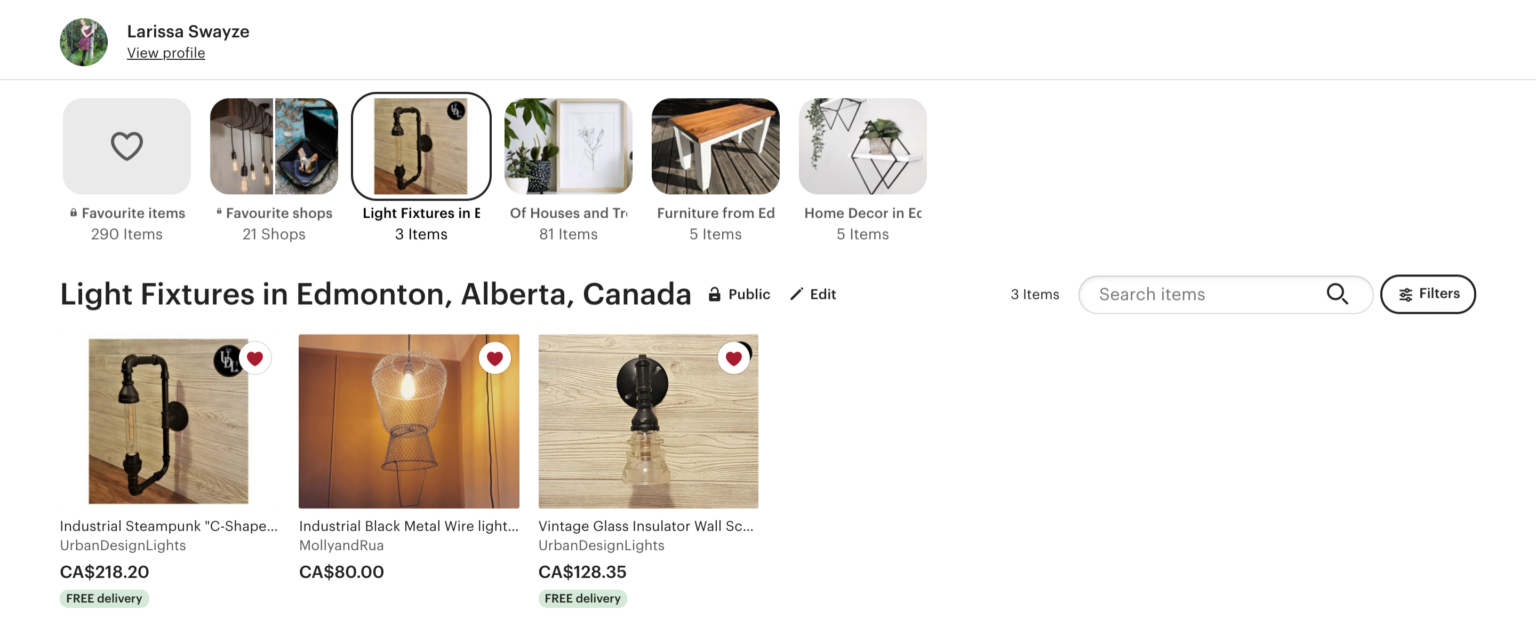The image is a screenshot of a website or app, characterized by a layout that is approximately three times wider than it is tall. At the top, there is a small profile picture of a woman dressed in maroon, though the details are hard to discern. Next to the image, her name, Larissa Swayze, is written in black text, accompanied by a black, underlined link titled "View Profile." The background of the entire layout is white. 

A horizontal gray line extends across the full width of the interface, dividing the upper and lower sections. The bottom section features multiple interactive squares with rounded edges, each representing a different category or clickable area, suggesting that this might be a shopping platform. The categories include "Favorite Items," "Favorite Shops," "Light Fixtures," "Houses and TR," "Furniture from Ed," and "Home Decor in Ed." Each category presumably contains various items.

Beneath these categories, there is another section titled "Light Fixtures in Edmonton, Alberta, Canada." This section appears to showcase three specific items, each with a listed price.